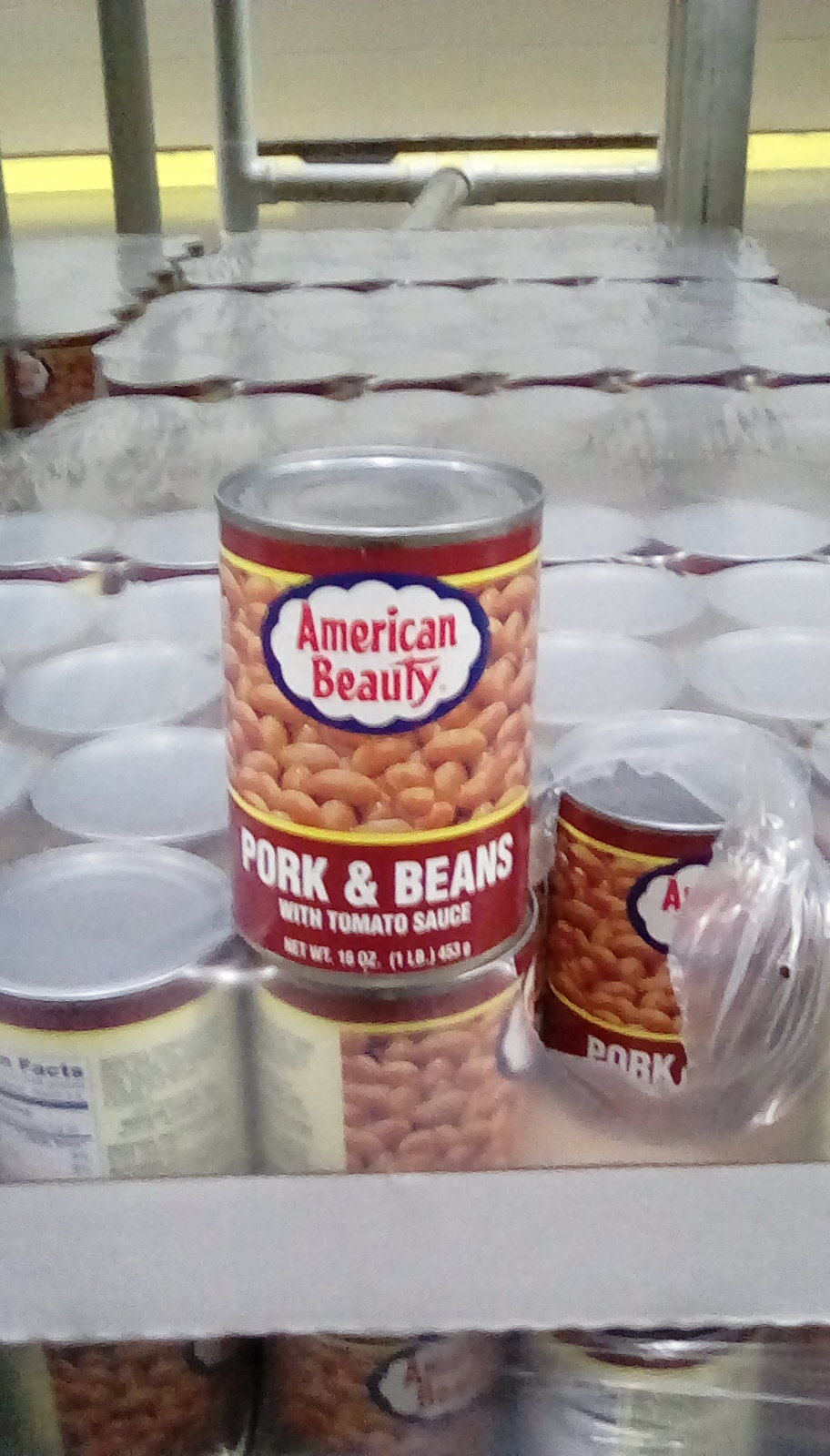The photograph showcases four rows of neatly stacked boxes containing canned pork and beans. The boxes, made from white cardboard, only rise halfway up the cans, leaving the upper portion of the cans exposed. Each can is wrapped in plastic for additional security. In the foreground, one box is open, revealing a single can resting on top.

The can itself is aluminum and notably lacks a pull ring. It features a maroon-colored label with the brand name "American Beauty" prominently displayed in vivid red letters. The design on the label includes an image of white beans, partially obscured by the brand name. Below the beans, the product name "Pork and Beans" is printed in white text, followed by the phrase "With Tomato Sauce," also in white text. Finally, the weight of the contents is noted at the bottom of the label. The overall scene emphasizes the product's branding and packaging while offering a glimpse into the organized storage of these canned goods.